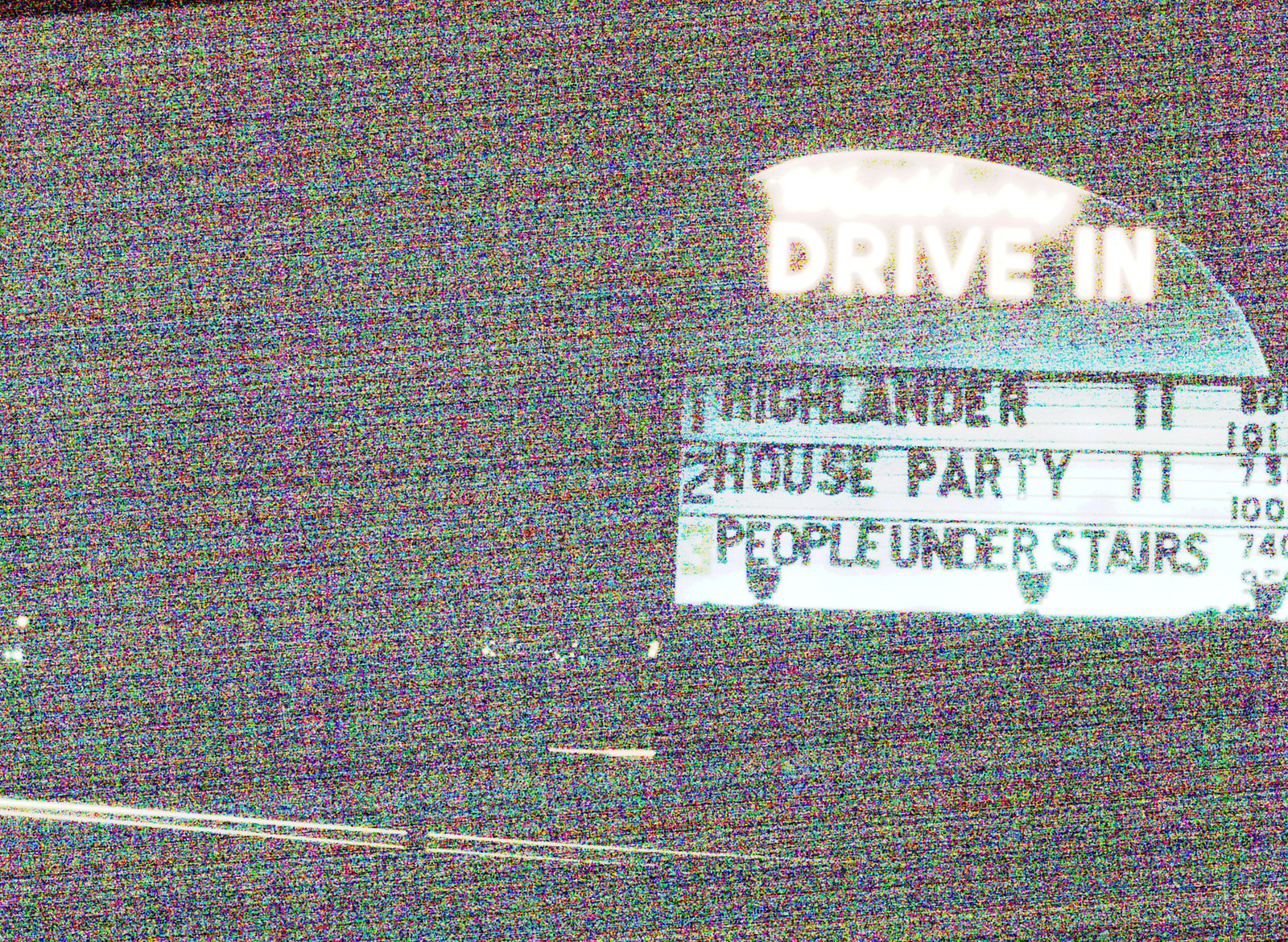This image depicts a heavily pixelated and staticky scene reminiscent of the colorful static often seen on old televisions. The screen is overwhelmed with myriad hues including reds, blues, and yellows, blending chaotically across the entire display. Amidst this background is a sign that reads "Drive-In" in bold white text. Below this sign, the titles of three movies are listed, albeit slightly obscured: "Highlander," "House Party," and "People Under the Stairs," presumably accompanied by their showtimes, though the latter details are partially cut off. Additionally, sporadic, flickering lights dot the screen, enhancing the retro, low-resolution aesthetic. Overall, the image primarily conveys the nostalgic experience of a drive-in theater through a vintage, pixelated lens.